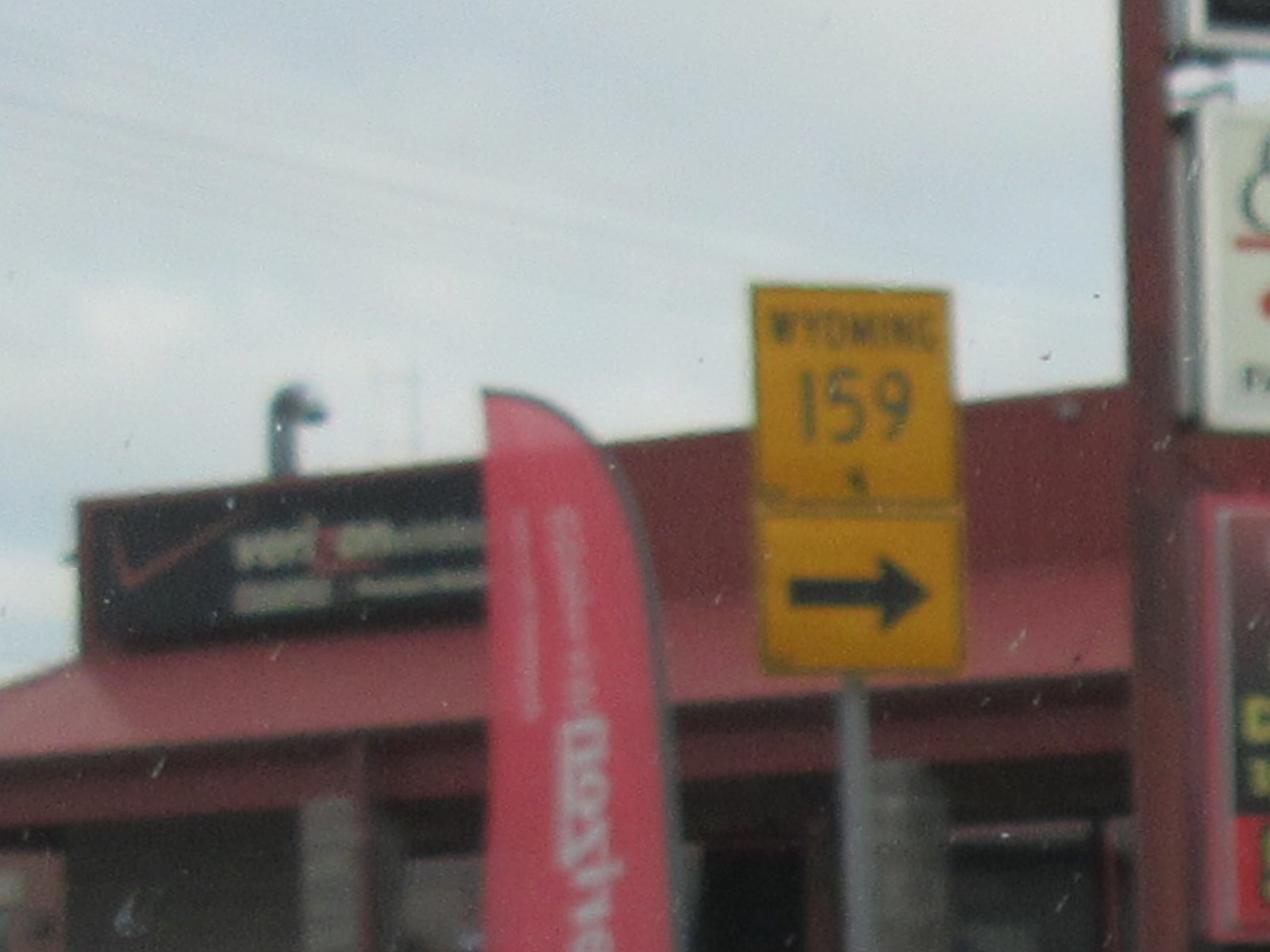The image depicts a blurry scene, likely taken through a dirty windshield, possibly from a car, which appears to be pulled up at a gas station. Central to the image is a building with a distinctive red roof and a black Verizon sign adorned with white lettering and a red checkmark. To the front left of this building is a red object with white print — potentially a flag or a snowboard. Prominently displayed is a yellow street sign on a silver pole that reads "Wyoming 159" in black letters, with an arrow pointing right. The scene includes another yellow sign of the same shade beneath the first, angled to the right. Additionally, there's a hint of a gas pump on the far right side. The sky above is overcast, rendered in a grayish-blue hue, and power lines are faintly visible, adding to the overall sense of desolation with no people present.